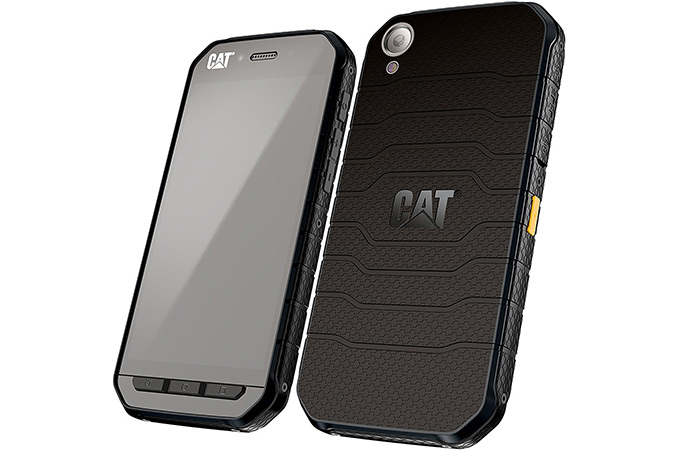The image showcases the design rendering of a CAT-branded mobile device and its cover. On the left, the front side of the device features the brand name "CAT" in white letters at the top left, set against a gray screen. The front has three black buttons at the bottom, and the device has flat corners rather than rounded ones. On the right, the back side of the device is displayed, highlighting a ribbed, rubberized black texture with "CAT" prominently in the middle in gray lettering, complete with a small triangle under the "A." The back also features a circular opening at the top left for the camera, a yellow or orange button along the right side, and additional details such as a small silver component, possibly a microphone, at the top. The images are taken at a slight angle, showing a bit of the right side of the device in both views.